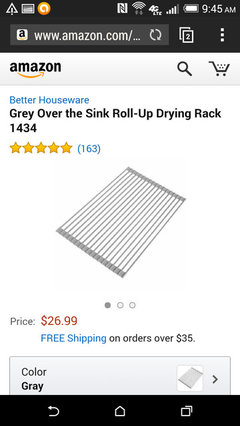This is a detailed description of a cell phone screenshot displaying an Amazon product page. At the top, the screen features a large black rectangle that contains various cell phone status icons in gray. Beneath this, a gray search bar is visible on the left side, featuring the Amazon logo, while to its right, the URL "www.amazon.com/" is displayed in white. Adjacent to the URL is a reload symbol, followed by the outline of two stacked boxes, with the top box containing the number "2." Further right, there is an ellipsis represented by three vertically stacked white dots.

Below this section, there is a light gray rectangle. On the left, the word "amazon" is written in bold, lowercase black letters, accompanied by the iconic orange Amazon arrow underneath. On the right side of the rectangle, there are gray icons for a magnifying glass and a shopping cart.

The main content of the screenshot begins with a white background. In the upper left-hand corner, the brand name "Better Houseware" is written in blue. Below this, a bold black title describes the product: "Gray Over-the-Sink Roll-Up Drying Rack." The item is identified by the number "1434." Underneath the title, five yellow stars indicate the product's rating, with the number "163" in blue within parentheses, denoting the number of reviews. Centrally positioned below this information is an image of the drying rack.

Further down, on the left side in gray text, the word "Price:" is displayed, followed by the cost of the item in larger red characters: "$26.99." Below the price, there is a note in blue indicating "FREE Shipping," and it specifies in gray that this applies to orders over "$35."